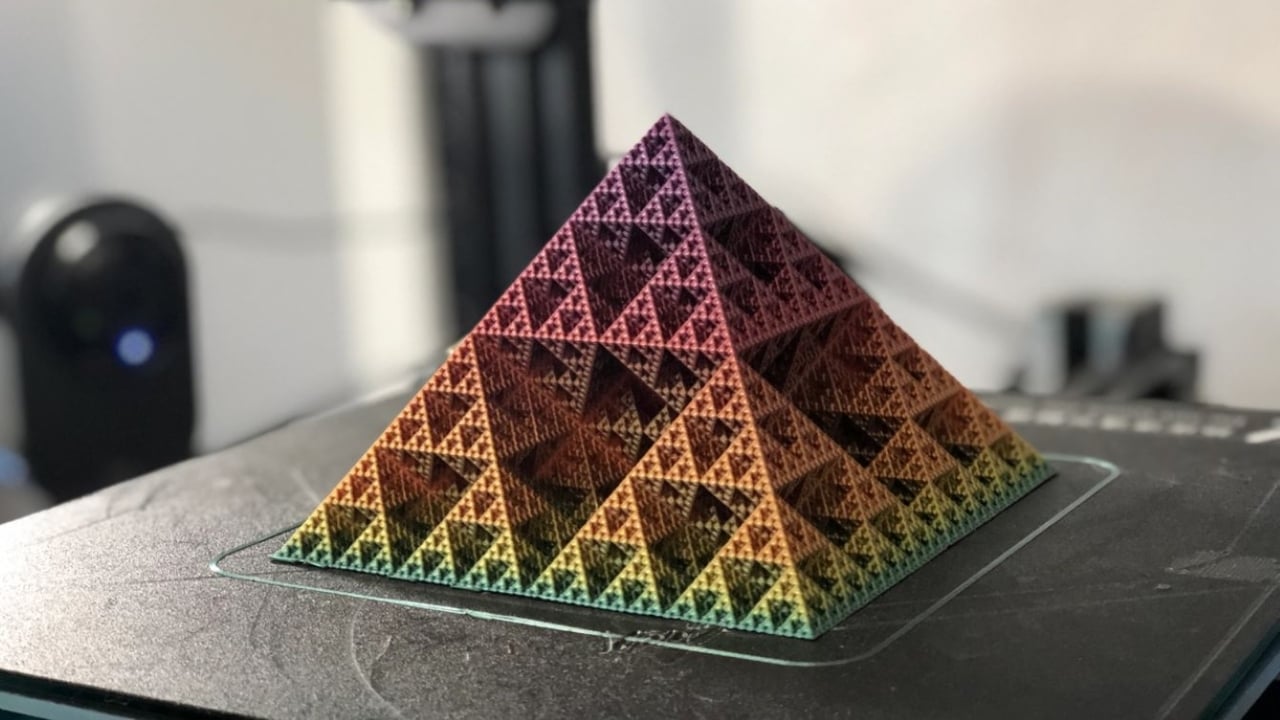This image features a horizontally aligned, rectangular photograph, primarily showcasing a colorful, intricately designed pyramid model. The pyramid, positioned centrally on a black, textured surface that might be a desk or a large book, captivates with its vivid color gradient transitioning from bottom to top: starting with an aqua green at the base, ascending through yellow, orange, and reddish hues, and culminating in a purple apex. Each side of the pyramid displays triangular cutouts within, some of which are black and vary in size, enhancing its detailed and possibly three-dimensional appearance. The black surface upon which the pyramid rests features what appears to be outlines drawn with glue. The backdrop is a blurry, white-walled space with indeterminate black objects, adding a context of an indoor setting, likely an art studio or a workspace. This composition, a blend of artistic creation and puzzling craftsmanship, invokes a nuanced perception that it could equally be a piece of art or a meticulously assembled puzzle.